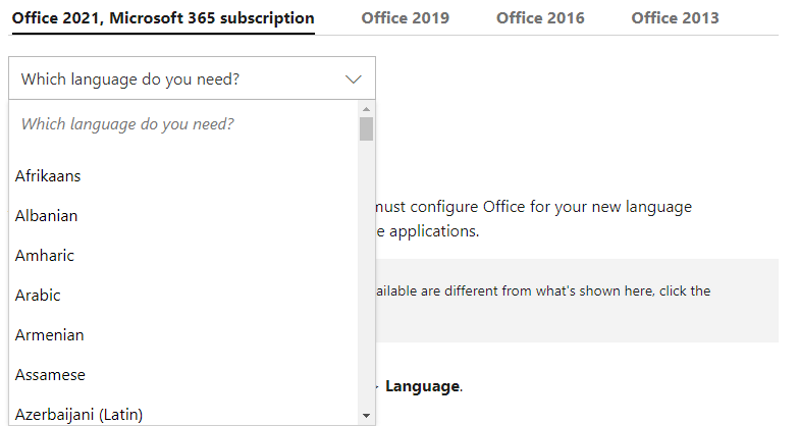The image depicts a web interface for Office 2021, specifically highlighting Microsoft 365 subscription options. Dominating the top section of the page, the words "Microsoft 365 subscription" are prominently displayed in bold black font. Beneath this header runs a solid black bar, which is visually connected to options for previous Office versions, namely Office 2019, Office 2016, and Office 2013.

To the left of the image, there is a prominently featured box labeled "Which language do you need?" accompanied by a dropdown menu. This menu allows users to scroll through and select their preferred language from a comprehensive list. The dropdown menu slightly overlaps a notification on the right-hand side of the page, which instructs users to configure Office for the selected language. The partial text visible suggests a step related to applications, although it is somewhat obscured.

Below the language selection box, another gray box contains truncated or partially obscured text, potentially indicating the availability of certain features or applications. The page also includes a standout label that reads "Language" in very bold, dark letters.

The overall appearance of this web interface is stark, with a monochromatic black-and-white color scheme, void of any additional color or icons. Most of the functional elements, including the language selection process, are clustered on the left side of the page. Users likely have the option to navigate between different Office versions such as 2019, 2016, and 2013, as needed.